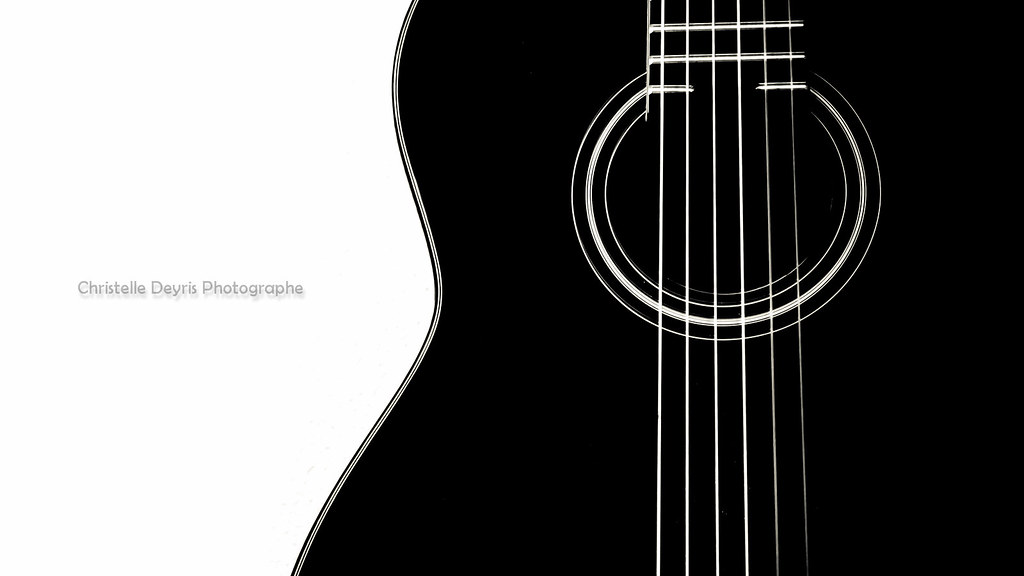The image showcases a clip art of a vertically oriented black guitar against a stark white background, covering the right three-quarters of the frame. The guitar's body, accentuated by a thin white outline on its left edge, features a prominent white concentric sound hole at its center. The six white strings appear darker and thicker on the left side, becoming progressively narrower and lighter toward the right. The guitar's fretboard is visible with three white frets before the image cuts off. On the far left side of the image, in very light gray letters, is the attribution: "Christelle Deyris Photography".